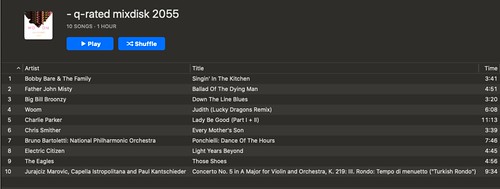This image showcases a playlist from a music streaming site titled "Q Rated Mix Disc 2055." The playlist's cover art is prominently displayed at the top. It features a collection of 10 songs, with the total duration of the playlist being approximately one hour. The interface includes blue play and shuffle buttons with white text for easy navigation.

Below the cover art, the playlist interface is organized into three columns: "Artists," "Title," and "Time." Each column lists the corresponding details for all 10 songs. The artists' names are listed under the first column, the song titles under the second, and the duration of each track under the third. The majority of the tracks have a runtime ranging between three to four minutes, with one notable exception lasting 11 minutes and 13 seconds.

The structured layout and detailed information provide users with a clear and concise overview of the playlist contents.